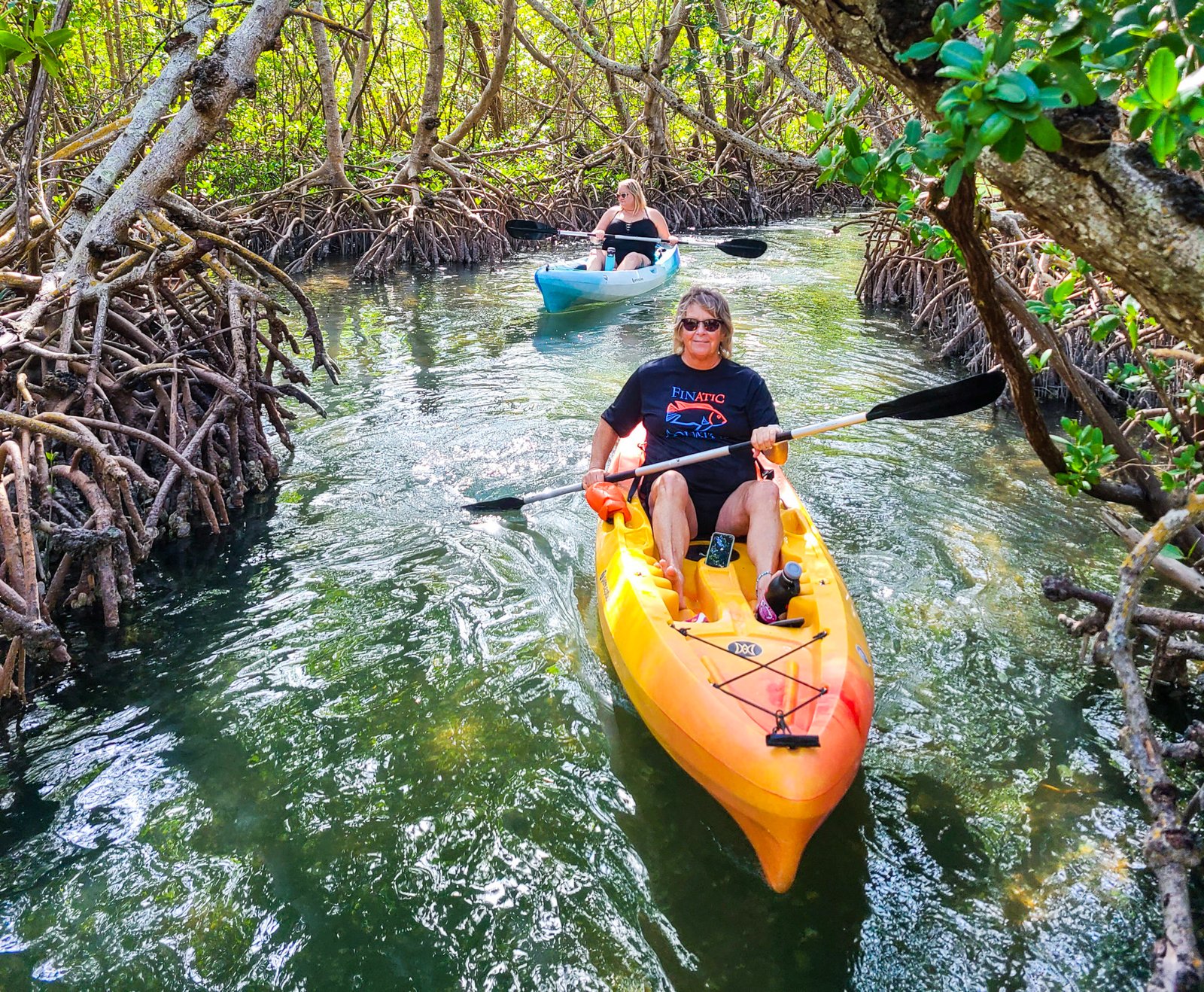The image captures a serene scene of two women kayaking through a lush, forested waterway flanked by dense mangrove trees. The water is a clear, almost lime-green color, suggesting a clean aquatic environment. In the foreground, one woman is seated in a yellow kayak, wearing a short-sleeved black T-shirt with the word "Fanatic" printed on it and sunglasses. She is holding a black paddle, her right hand dipping it into the water while her left holds it aloft. Behind her, a blonde woman paddles a light blue and white kayak and is dressed in a black bathing suit. Both kayakers are navigating through a narrow, almost jungle-like canal, surrounded by the exposed roots and thick greenery of the mangrove trees that cluster on both sides and extend into the background, creating a captivating, natural tunnel of foliage and light.